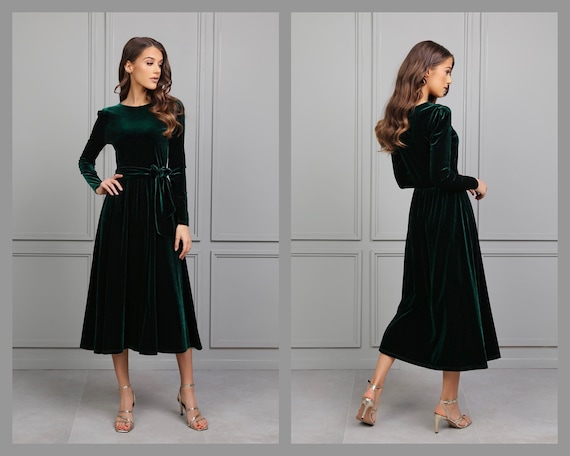The adjacent images depict a fashion catalog shoot featuring a woman modeling the same outfit from two different angles. In the left image, she stands facing forward with her head turned to the left, allowing a partial profile view. She dons silver sandals and a long-sleeved dress that falls just below the knee, equipped with shoulder pads, a round collar, and a belt detail at the waist. Her long brown hair cascades over her left shoulder, complementing the sophisticated look. The backdrop consists of a gray paneled wall that matches the gray floor, providing a neutral yet elegant setting.

In the right image, the woman maintains the same attire but is captured from a rear angle. She twists her torso so her back faces the camera while her head turns to the right. This pose highlights the silver heels of her sandals and offers a different perspective on the dress's fit and design details. The consistent gray background and flooring create a cohesive and classy visual frame for both images.